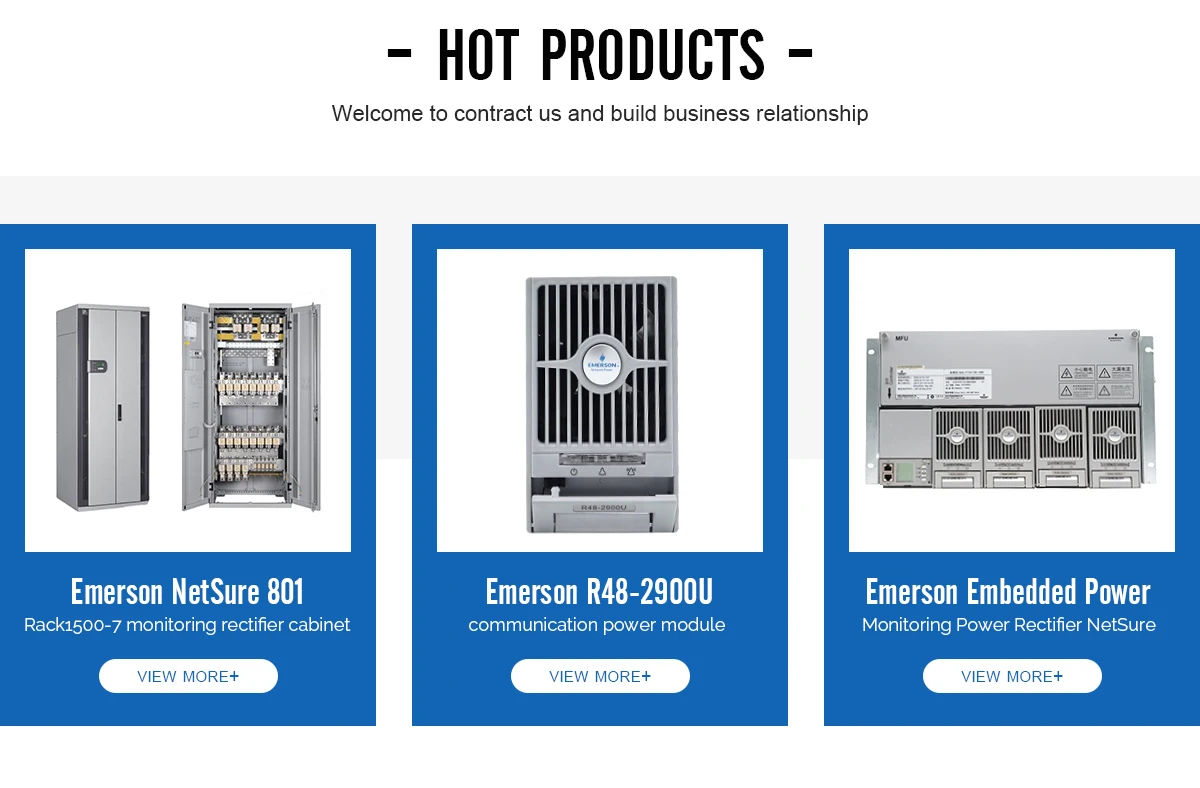The image showcases an advertisement or flyer for electronic devices, prominently titled "Hot Products" at the top. The ad invites viewers to contact the company to establish business relationships. 

Below the title, three separate images display different power supply products, each with detailed descriptions:
1. On the left is the Erminson Netsure 801.
2. In the center is the Erminson R48-2900U, identified as a communication power module.
3. On the right is the Erminson Embedded Power Monitoring Power Rectifier Netsure.

All three devices are horizontally aligned and share a sleek, silver coloration. The flyer provides an option to "View More" for additional information. The products seem to include a mix of power supply packs and a power module inside a cabinet-like structure, all designed for technical and logical applications.